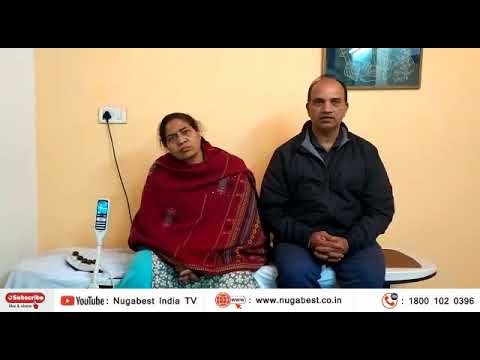This is a detailed image showing an East Indian couple, likely in their 50s to early 60s, seated together on what appears to be a narrow hospital bed or bench. The woman is on the left, wearing a cranberry-colored shawl with gold and violet accents, draped over a teal skirt adorned with a green and white floral pattern. Her hair is pulled back, and she holds what looks like a hand controller to the bed, suggesting she might be in a hospital setting. The man is on the right, dressed in a dark, thick black jacket with a gray lining and blue pants, displaying a deep receding hairline. Both have dark features and are looking straight at the camera. 

Behind them is a pale yellowish-beige wall with a black plug connected to a white electric outlet on the left, and a brown-framed photograph partially visible at the top right. The image appears to be a still from a video or broadcast, with a YouTube banner at the bottom displaying "YouTube NugaBest India TV," a website (www.nugabest.co.in), and a phone number (1-800-102-0396). The entire image is framed with narrow black borders at the top and bottom.